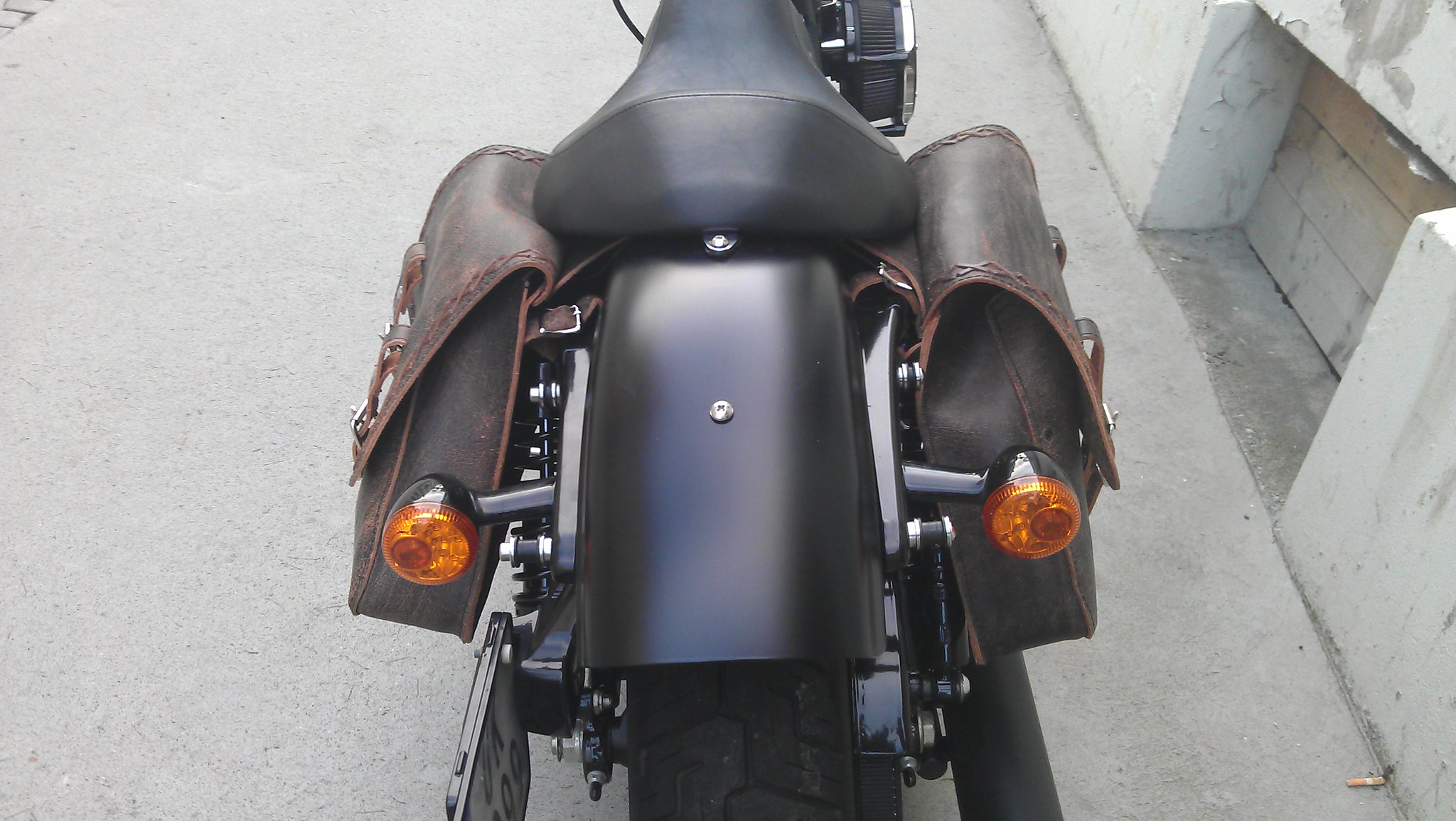This image is a close-up of the back end of a motorcycle parked in a paved alleyway with a gray wall on the right side. The motorcycle's black and silver frame prominently features a black seat, black fender, and partially visible rear wheel and gears. Two dark brown leather satchels are mounted on either side of the seat, secured with buckles and featuring clasps for closure. The motorcycle also displays orange blinker lights used as taillights. In the background, the gray wall has a square-shaped recess at the bottom that has been boarded up, adding a unique urban element to the scene.